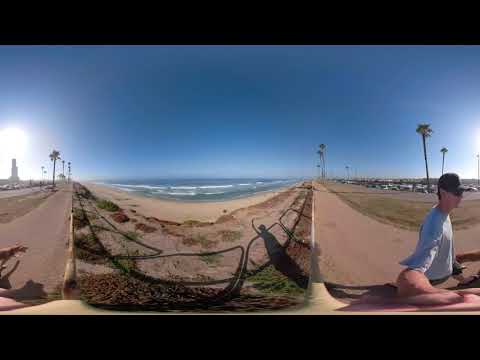The image captures a distorted, fisheye view of a beach scene, prominently featuring a man using a selfie stick. The perspective creates a three-section divide with the central part curved inward. The man, who is wearing a gray short-sleeve shirt, a black hat, and sunglasses, appears both in the far right and far left segments due to the distortion. He is walking along a sidewalk or dirt path near the beach, with multiple green and reddish ornamental plants lining the area. Palm trees with green leaves are scattered throughout, both in the foreground and background, which resembles a Southern California landscape. The ocean is visible in the distance, with waves crashing against the shore, and the sky above is vividly blue with the sun shining brightly. Black framing is present at the top and bottom of the photo, adding to the unique VR-like experience.